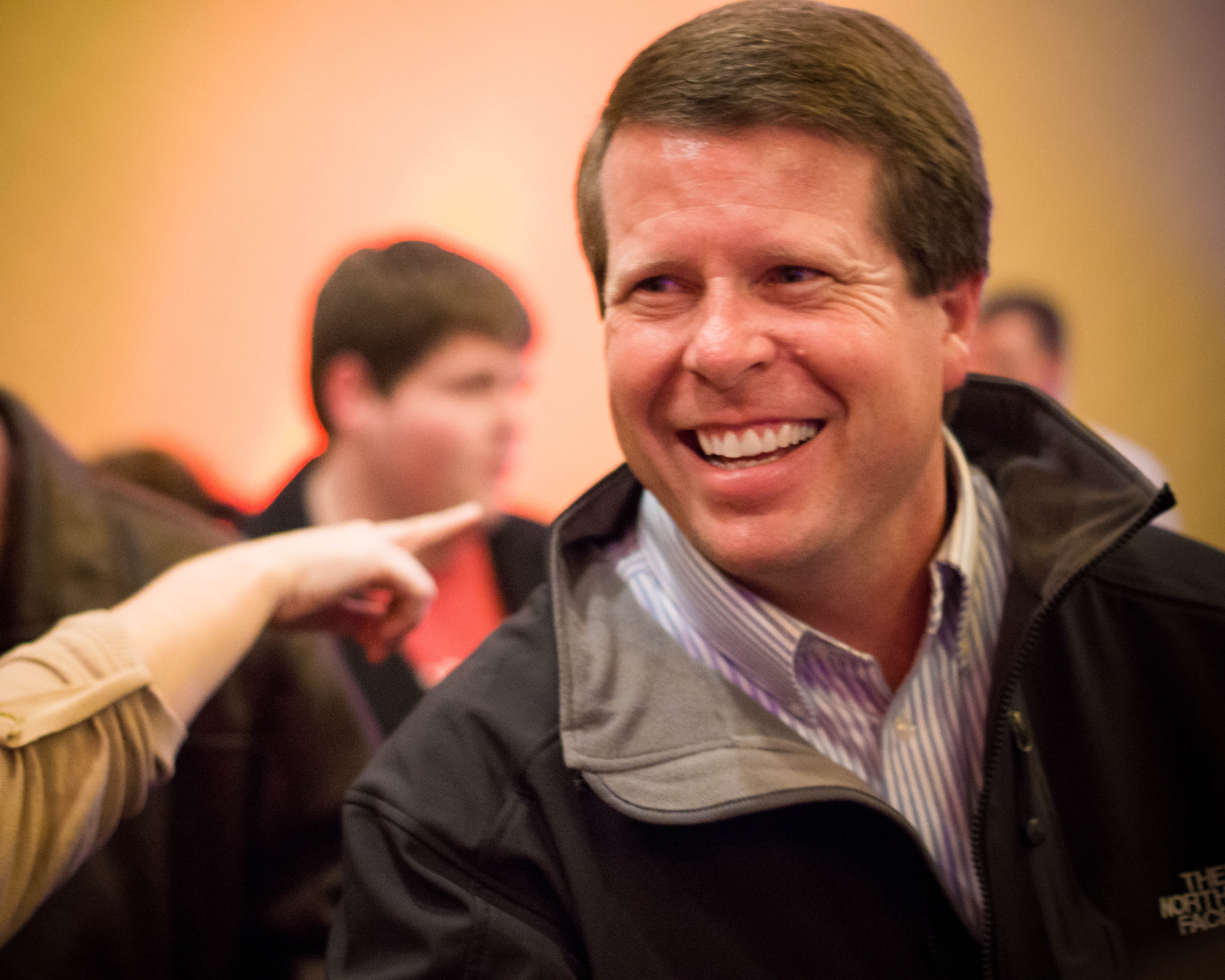The image features reality TV star Jim Bob Duggar from "19 Kids and Counting," positioned on the right side. He is smiling broadly, showcasing both his top and bottom teeth, with little wrinkles forming at the corners of his eyes. His hair, combed neatly to the side, is brown. Jim Bob is wearing a black zippered jacket with "The North Face" logo on the left chest area, and underneath, he has on a collared shirt with white and gray, or possibly blue, stripes.

Next to Jim Bob on the left, there is a female figure wearing a brown shirt, though only her arm is visible. Behind Jim Bob, another man with short brown hair is seen wearing a red t-shirt and a black jacket. Further in the distance, there is another male figure with short brown hair, and the backdrop appears to be yellow but somewhat blurred, creating a sense of depth in the image.